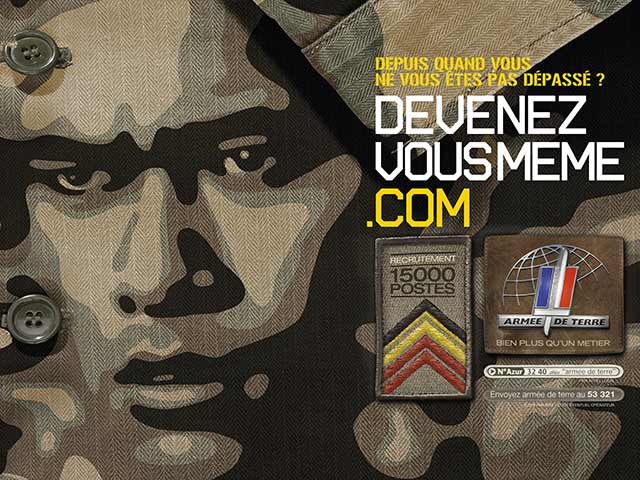The image appears to be an advertisement for a French army unit. On the left side, there's an artistic rendering of a soldier's face created using a camouflage pattern, along with two buttons which are part of a uniform. Additional elements include a military patch displaying black, yellow, and red chevrons. The right side of the advertisement contains text in French, starting with "DEPUIS QUAND VOUS NE VOUS ETES PAS DEPASSE?" and prominently features the call to action in large white letters, "DEVENEZ VOUS METS." Beneath the text, there are smaller, possibly unreadable, patches or advertisements related to recruitment and website information like "DEVENEZ.COM."